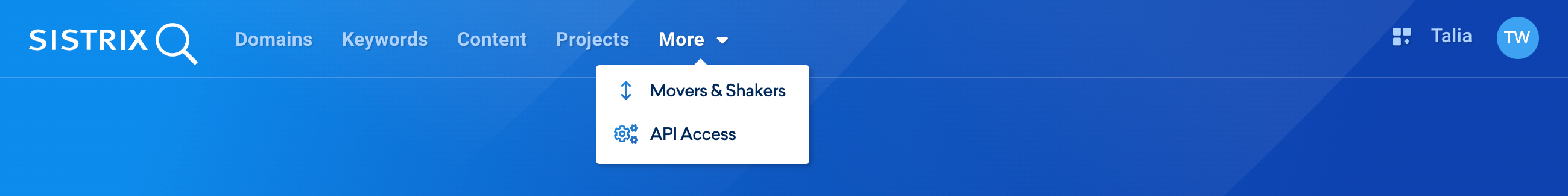This screenshot appears to be a small, highly detailed depiction of a web-based application or software program with a predominantly blue color scheme. The gradient background transitions from a lighter blue on the left side to a darker blue on the right. The company's name, "Synthstrix," is prominently displayed in the upper-left corner, followed by a magnifying glass icon that likely serves as a search function.

Below the company's name, there are several navigational tabs organized in a row: "Domain," "Keywords," "Content," "Projects," and a "More" tab which has an error icon next to it. The current view in the screenshot is under the "More" tab, specifically showing options labeled "Movers and Shakers" and "AP Access."

The top-right section of the interface features three distinct icons. The first icon consists of three small squares arranged in a grid, potentially representing additional settings or features. To its right, the name "Talia" is displayed, indicating the logged-in user. Further to the right, there's a circular icon with the initials "TW," presumably representing the user's profile picture.

Text throughout the interface is rendered in white and gray colors, offering a clear contrast against the blue background. A horizontal line divides the middle of the screen, suggesting sections or modular components of the program. The overall design and elements hint that this is likely a tech company application designed for professional or work-related tasks.